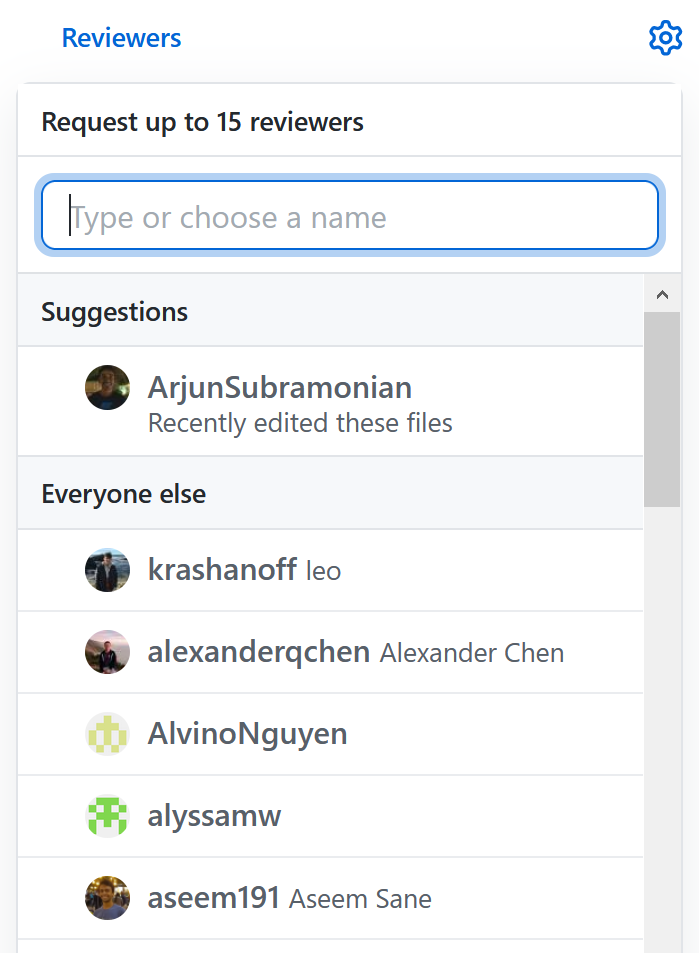The image showcases a website interface. At the top of the page, the title "Reviewers" is displayed prominently in blue text. On the right side, a blue cog icon is situated, suggesting settings or configuration options. Below the title, there's a rectangular section with a white background that reads "Request up to 15 reviewers" in either blue or black text, with the number "15" shown numerically. 

Beneath this section is a search bar outlined in blue, accompanied by the placeholder text "Type or choose a name." Further down, there is a gray background section labeled "Suggestions" in black text. Here, it mentions that "Arjun Subramanian recently edited these files," and displays an avatar image in a circle to represent this user.

Following this, a list of five suggested reviewers is shown, each accompanied by a circular user image. The list includes:
1. Crash and Off Leo
2. Alexander Q. Chen (also listed as Alexander Chen)
3. Alvino Nguyen
4. Alyssa M.W.
5. Aseem191 (identified as Aseem Sain)

Each entry mirrors the format of displaying the user's avatar alongside their name, reinforcing the platform's focus on visual and textual information for user identification.